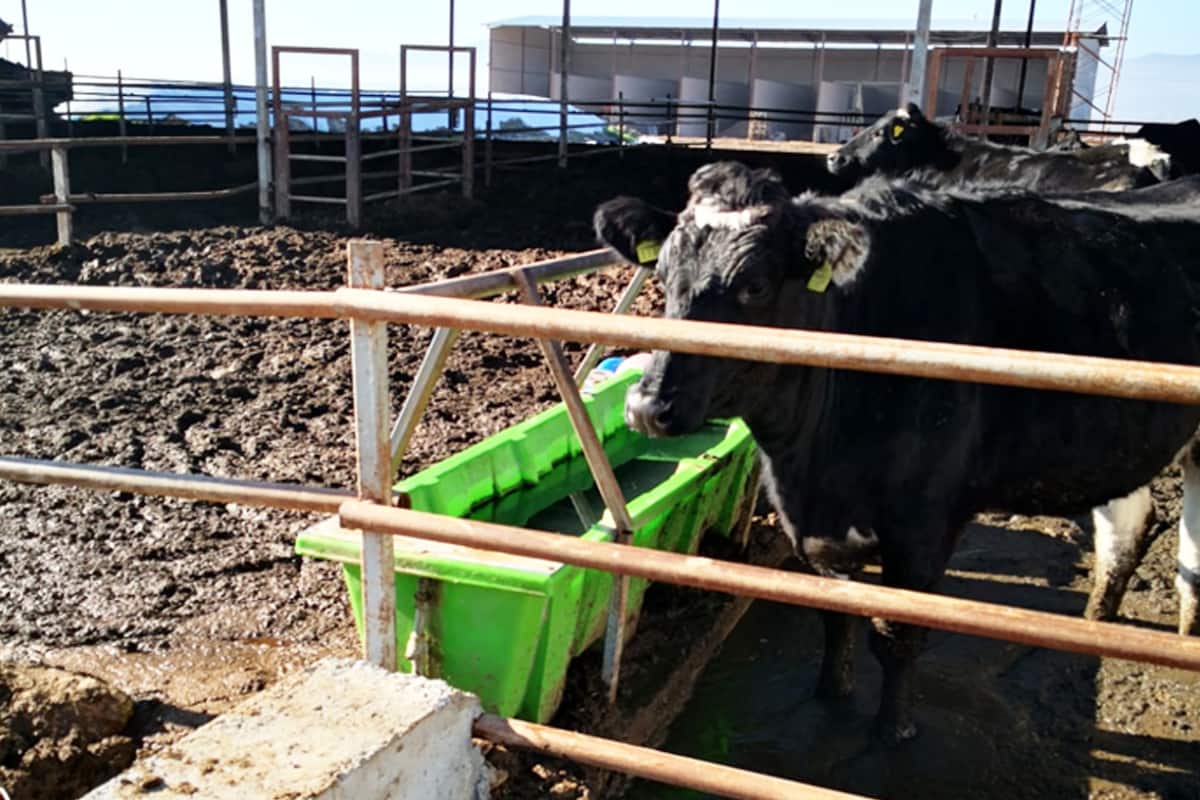The photograph depicts a holding pen divided into two sections, constructed with slightly rusty steel pipe fencing. In the right section of the pen, two predominantly black cows with white spots are standing on wet, muddy ground. The cow in the foreground, which has a white patch on its forehead and two yellow tags in its ears, is facing three-quarters towards the camera. The second cow is positioned in the background, facing left and not looking at the camera. A green plastic water trough with slightly brown water is situated centrally in front of them. The adjacent left section of the pen is empty, featuring a very muddy surface. Surrounding the pen, there is an extensive network of piping, and an open-sided building with stalls, possibly milking stations, is visible in the background.